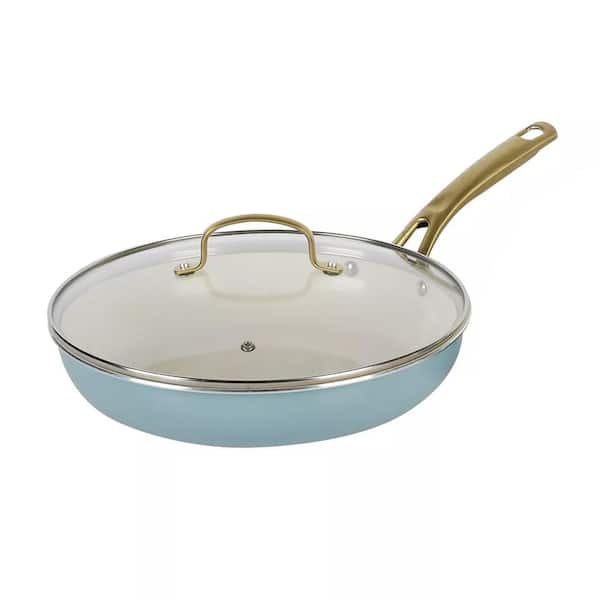This image is a highly detailed color photograph of a non-stick ceramic-coated frying pan with a matching glass lid, set against a clean, white background. The frying pan itself boasts a sleek Carolina blue exterior, while the interior presents a contrasting white surface. The interior is minimally adorned with two silver rivets where the handle attaches. The handle, extending to the right and rear from the viewer's perspective, is made of sturdy metal and features a convenient hanging cut-out hole at the end.

The accompanying glass lid is slightly domed and framed with a chrome or steel rim, enhancing its durability and aesthetic appeal. Instead of a conventional central knob, the lid is equipped with a distinctive drawer pull-style loop handle, also chrome-finished, which curves gracefully and is securely attached with screws. Additionally, the lid incorporates a small vent hole for steam release, ensuring optimal cooking conditions. The detailed design elements highlight both the practical functionality and the elegant style of this frying pan, making it a versatile and attractive addition to any kitchen.